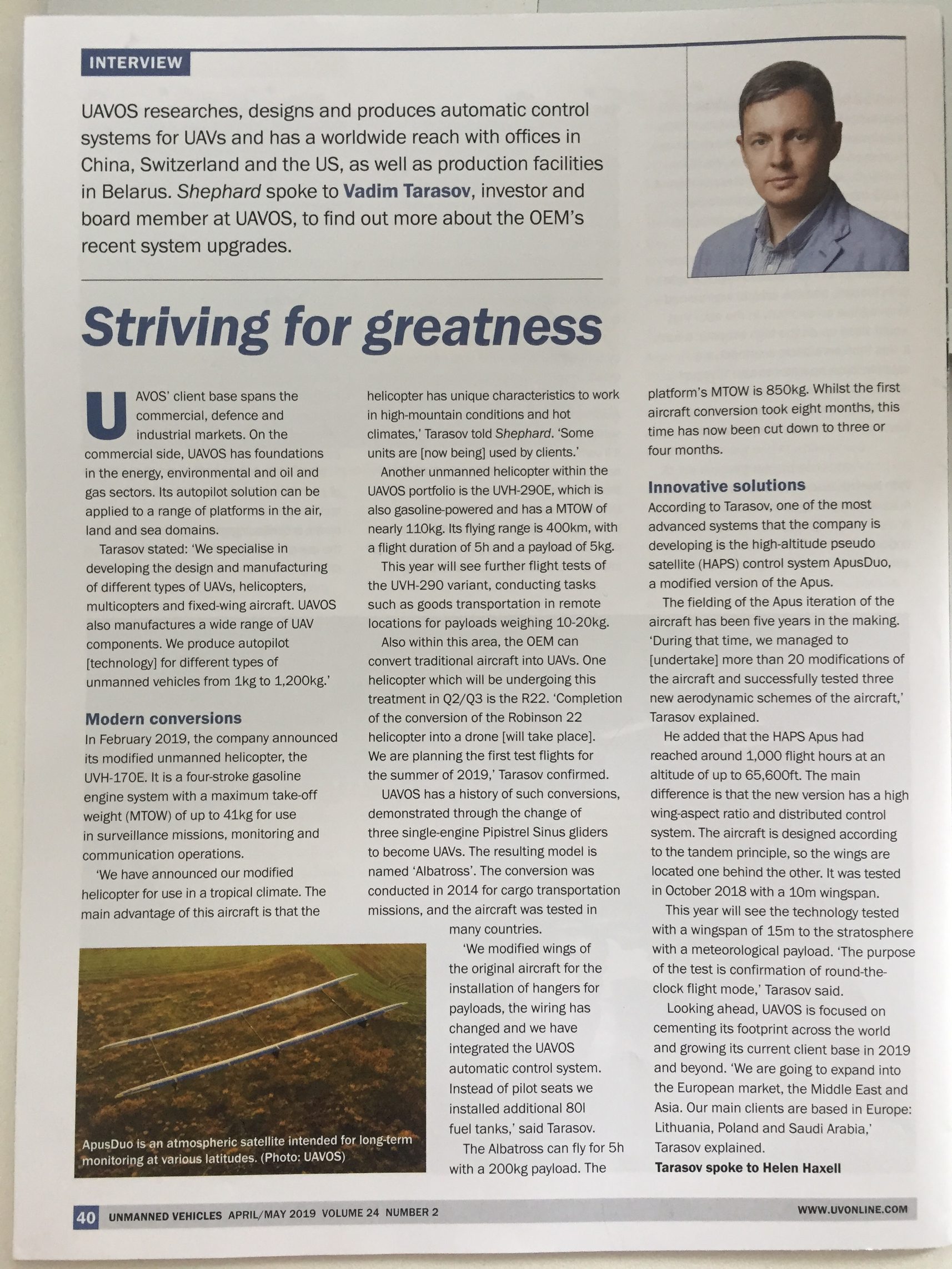The photograph, captured in portrait mode, features a magazine article situated on a cream-colored surface. The upper left-hand corner of the image reveals a snippet of the background, confirming that it is not a screenshot. Positioned prominently on the right-hand side, we can observe the edge of the magazine.

In the bottom-left corner of the magazine cover, housed within a purple square, is the number "40". The background is gray, and the cover text reads: "Unmanned Vehicles April/May 2019, Volume 24, Number 2". Additionally, the website "www.uvonline.com" appears on the right-hand side.

The content of the article is introduced at the upper left-hand corner, where the word "Interview" is written against a blue background. The main headline states: "UAVOS researches, designs, and produces automatic control systems for UAVs and has a worldwide reach with offices in China, Switzerland, and the US, as well as production facilities in Belarus. Shepard spoke to Vadim Tarasov," highlighted in blue, "an investor and board member at UAVOS to find out more about the OEM’s recent system upgrades."

To the right of the text, there's an image likely belonging to Vadim Tarasov. He has light skin, short brown hair, and is dressed in a blue button-up shirt paired with a light blue jacket. Just above his image, in dark blue text, is the phrase "Striving for Greatness".

The article is organized into three columns:
- The first column features the section title "Modern Conversions" highlighted in blue.
- The second column does not have any highlighted sections.
- The third column includes another highlighted title, "Innovative Solutions," and mentions at the bottom: "Tarasov spoke to Helen Haxel."

Lastly, at the bottom of the layout is an image of a satellite, rounding out the visual and textual elements of this detailed magazine article.